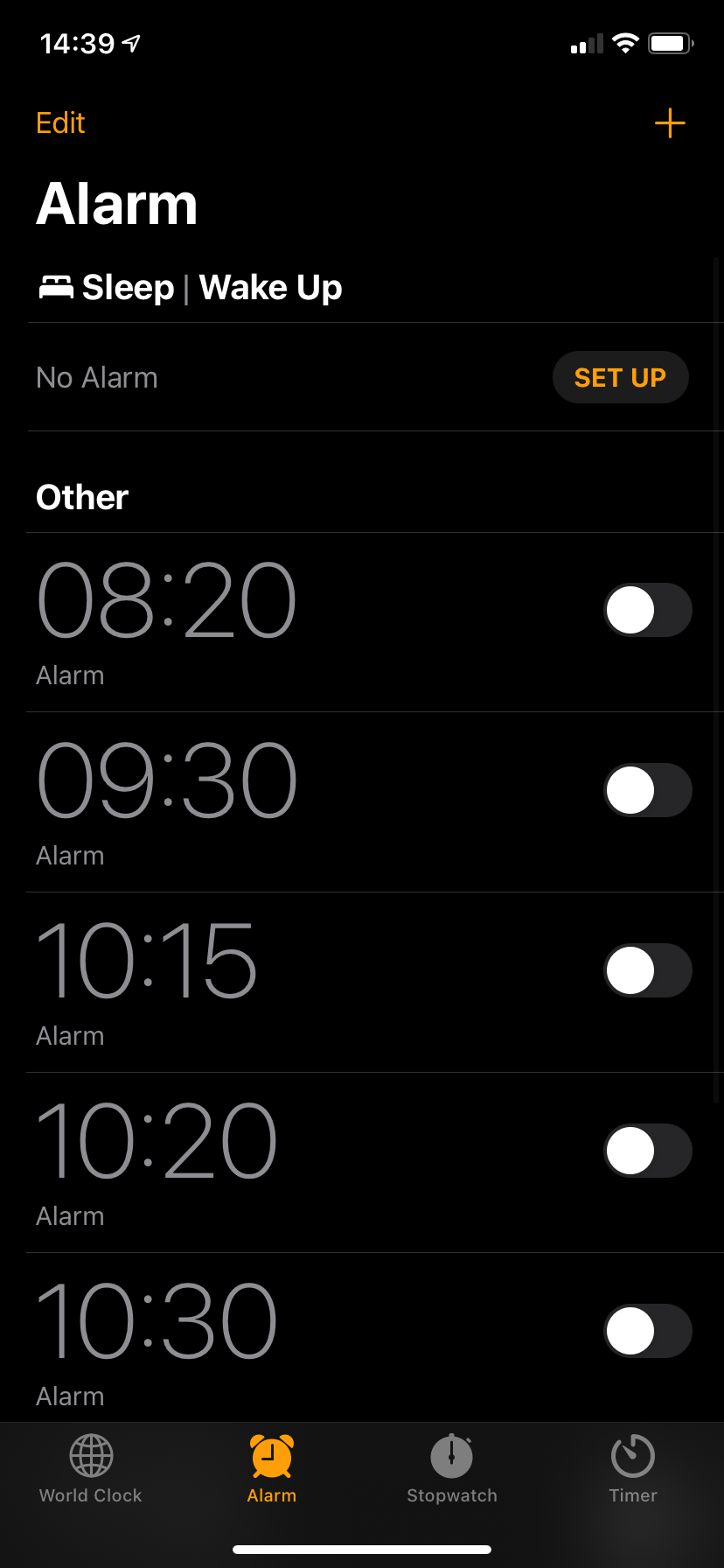A screenshot of a phone's alarm app interface with a sleek black background, accented with white text and orange buttons. At the top of the screen, the current time reads 14:39 and the battery is nearly full at 97%. Below the status bar, an orange "Edit" button is positioned on the left, and an orange "+" button is on the right, indicating the options to modify or add alarms. 

The main heading "Alarm" confirms the active tab, followed by a secondary section titled "Sleep | Wake Up" which currently shows "No Alarm". To the right of this is an orange "Set Up" button, inviting users to configure a new wake-up schedule. The central portion of the screen lists preset alarms under the section "Other." The alarms are set for 08:20, 09:30, 10:15, 10:20, and 10:30, all of which are currently toggled off with switches on the right side.

At the bottom of the screenshot, there are navigation buttons for different features of the app: "World Clock," "Alarm" (which is highlighted to show the current screen), "Stopwatch," and "Timer."